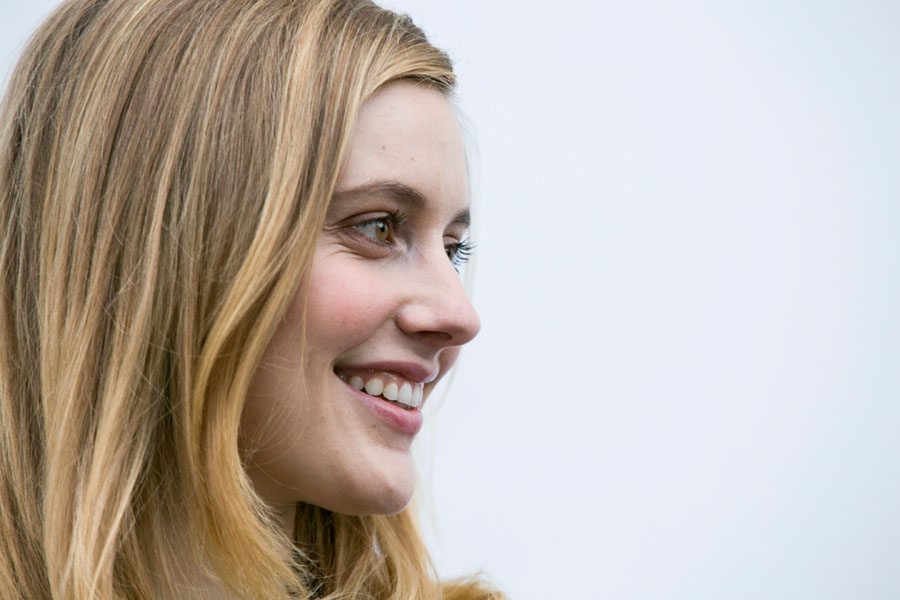The photograph features an attractive woman with long, cascading blonde hair. Positioned on the left side of the image, she faces to the right, her expression adorned with a radiant smile that highlights her nice teeth and lightly applied lipstick. Her olive, or possibly light brown, eyes add to her captivating appearance. The image captures her from around her neck to the top of her head, emphasizing her face, flowing hair, and part of her shoulders. Set against a light baby blue or gray background, the composition employs significant negative space on the right, accentuating her sideways glance. The overall style suggests she might be an actress, but she remains unrecognized.